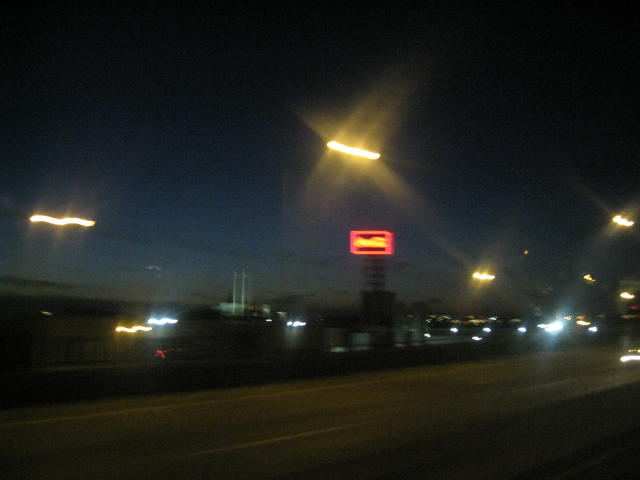This nighttime photograph, likely captured from the side window of a moving car on a highway, depicts an urban scene with a palpable sense of motion. The camera's position suggests it may be taken from the back seat, directed toward the left lane. The image features a cityscape in the distance, blurred by the motion and low light conditions. The night sky is a deep navy blue, contrasting against various lights from street lamps, buildings, and vehicles.

Prominent in the composition is a billboard in the distance with a red border and yellow text, reminiscent of a Coca-Cola advertisement, though the exact branding is indiscernible due to the blur. The scene also includes street lamps, whose lights appear as squiggly streaks due to the camera's motion. The highway itself shows two lanes separated by a middle concrete barrier, and while no cars are visible in the opposite lane, the tangled lights of passing vehicles in the foreground create a dynamic, chaotic pattern. The photo, encompassed mostly in shades of gray accentuated by yellow, red, and white lights, conveys a sense of bustling urban movement captured in a fleeting, impressionistic moment.